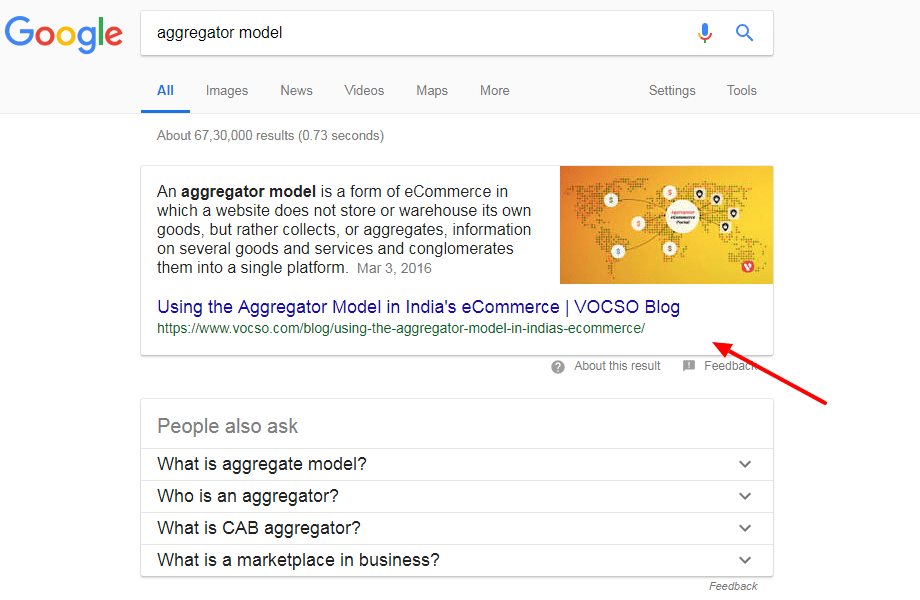A screenshot of a Google search page shows various elements clearly. At the top left corner, the iconic Google logo is displayed with each letter in a different color: blue, red, yellow, blue, green, and red. Below the logo is a white search bar containing the text "Aggregator Model." To the right of the search bar, a microphone icon and a magnifying glass (search icon) are visible.

Beneath the search bar, there's a navigation menu with tabs labeled "All," "Images," "News," "Videos," "Maps," and "More." The "All" tab is underlined in blue, indicating it is currently selected. Further to the right are options for "Settings" and "Tools."

The page features a snippet at the top that provides information on an aggregator model for e-commerce. This model does not store or warehouse its own goods but instead aggregates information about various goods and services, presenting them on a single platform.